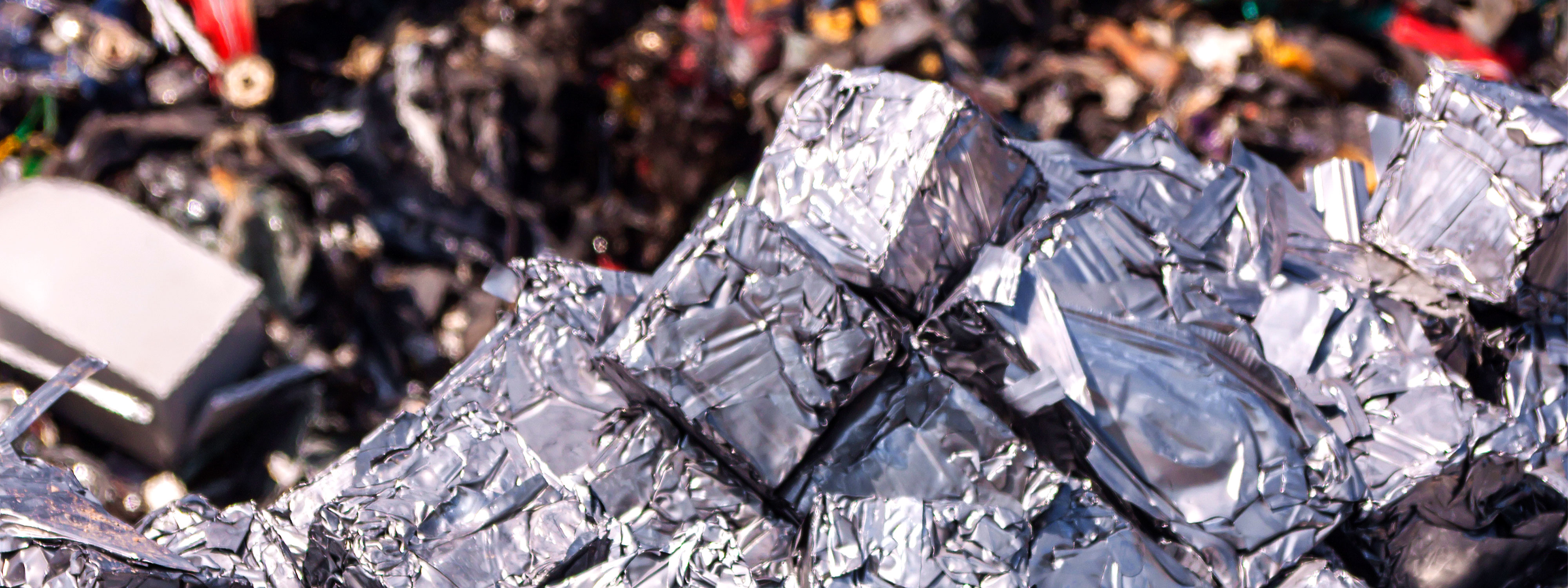In the foreground of the image, there is a large, irregular mass of what appears to be melted and fused aluminum or tin. This metallic clump, resembling metal slag, is composed of numerous small cubes and rectangles melded together, extending from the lower left to most of the right side of the image. The surface of the metals reflects sunlight, showing a grayish hue with a textured appearance marked by pits and lines which suggest high-temperature forging and cooling. 

Centered towards the right side of the image, these metallic forms are reminiscent of crushed and condensed aluminum, likely sourced from scrap materials such as pop cans. The background is filled with indistinguishable, blurred objects that hint at a setting like a landfill or junkyard, adding to the chaotic and cluttered atmosphere. 

Among these blurred items, a gray box touches the left-edge, and the middle-left portion of the image features an ambiguously shaded area with hints of red, brown, orange, and white scattered especially in the center and upper right sections. There's also a notable brown patch slightly left of center, and a metal rod can be discerned above a red object with a brown circle and black dot. The overall scene appears to be taken on a sunny day, emphasizing the reflective quality of the aluminum and the jumbled nature of the background items.